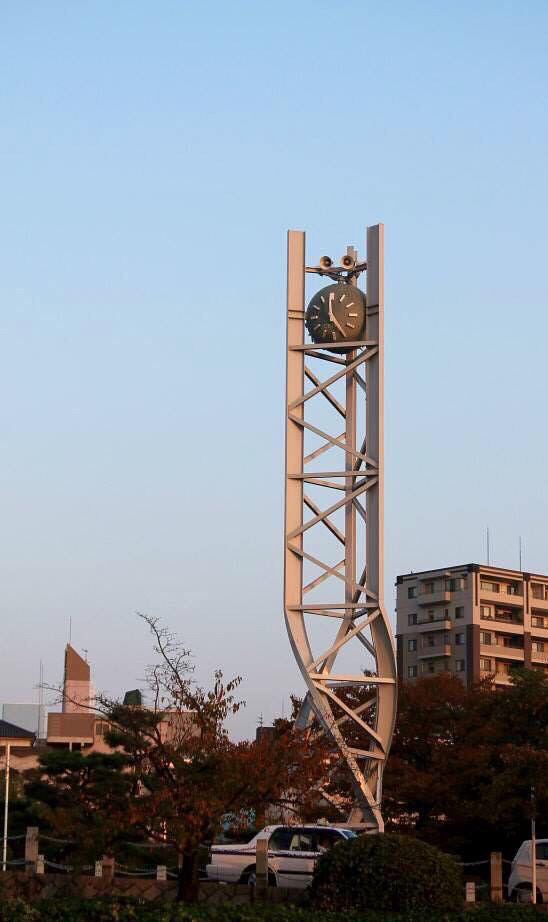The image features a striking gray twisted metal sculpture, likely made of steel, that dominates the scene. The base of the sculpture is a spiral, reminiscent of DNA, before extending straight upwards. The structure is laden with diagonal and horizontal beams for support and stands about two-thirds the height of the photo, towering over 50 feet. At the very top, encased within the supporting structure, is an analog clock with Roman numerals, showing approximately 12:25. Above the clock, there appear to be two speaker-like objects.

Below the sculpture, a white car with possible blue detailing is parked in a lot, separated from the camera by a chain-link fence. Surrounding this area are several trees and bushes, including one to the left and several behind the car, adding splashes of green. In the distance, a multi-floor apartment building with balconies and spire-like antennas is visible, while more nondescript buildings loom to the left. The scene unfolds beneath a clear blue sky, suggesting it's a pleasant day.